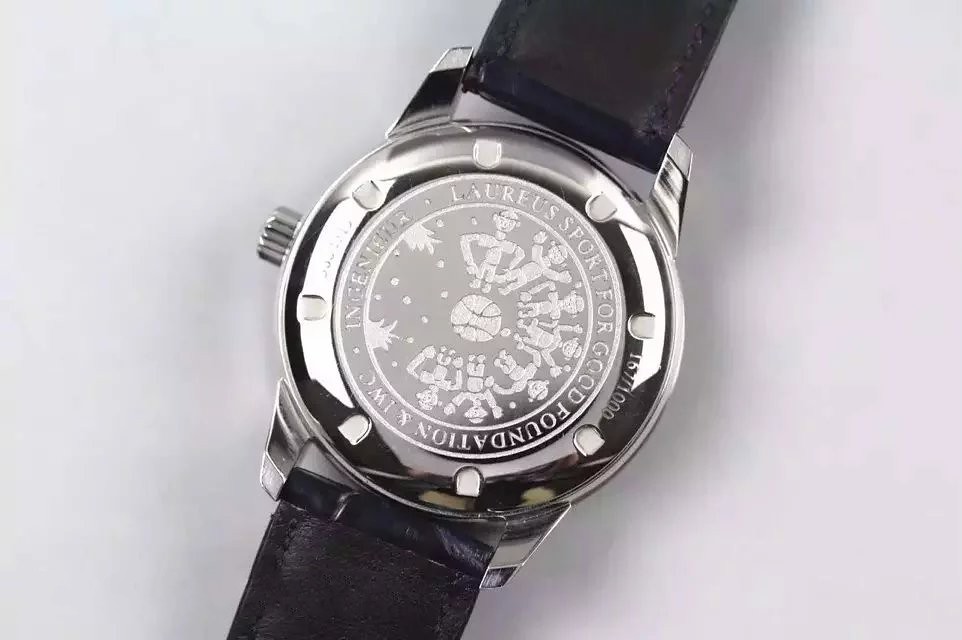In this photograph, a sophisticated wristwatch is displayed with its backside facing up. The entirety of the watch case is crafted from polished silver, exuding a sense of elegance and refinement. The watch features black leather straps, which are also visible, adding a classic touch to the overall design. The watch is thoughtfully positioned on a pristine white background, allowing its details to stand out.

The crown, or the small winding knob, is positioned on the left side of the watch, adding a unique aspect to the design. The most striking feature of the image is the intricate carvings on the back of the watch. At the center, there is a relief resembling a basketball, flanked by detailed engravings that look like small figures, adding an artistic and thematic element to the watch.

Surrounding these carvings, inscriptions are meticulously etched into the silver surface. Prominently displayed is the text "Loris Sport for Good Foundation" along with the well-known luxury watch brand "IWC." However, there is another word engraved which remains indistinct and unreadable in this image. The overall presentation highlights the craftsmanship and the thematic resonance of the watch, celebrating both sport and luxury in a refined manner.